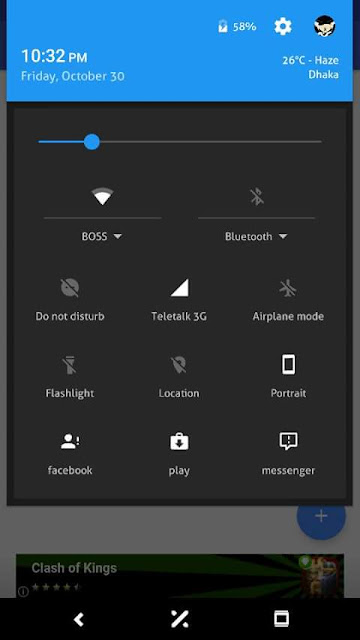The image shows a smartphone screen with a black background displaying various system settings and notifications. At the top, a status bar displays the time "10:32 p.m.," the date "Friday, October 30th," and the battery level at "85%." The temperature is shown as "26°C" with the condition "haze" in Dhaka, all in white font against the black background.

Below the status bar, there is a horizontal slider mostly positioned to the left with the draggable ball in blue, indicating it is part of an active setting. The left side of the slider is blue, while the right side is gray.

Under the slider, there is a dropdown menu titled "boss." Above it are Wi-Fi and Bluetooth icons with respective dropdown menus showing connection statuses. Three rows of three icons each are displayed below these:

- The first row includes "Do Not Disturb," "Tele Talk 3G," and "Airplane Mode."
- The second row includes "Flashlight," "Location," and "Portrait."
- The third row shows "Facebook," "Play," and "Messenger."

The bottom part of the screen appears to be semi-transparent with a gray tint, overlaying a white background. Partially visible here is text indicating the popular game "Clash of Kings."

Overall, the smartphone screen seems to be on a settings or quick access menu with a notification from "Clash of Kings" peeking through from behind.